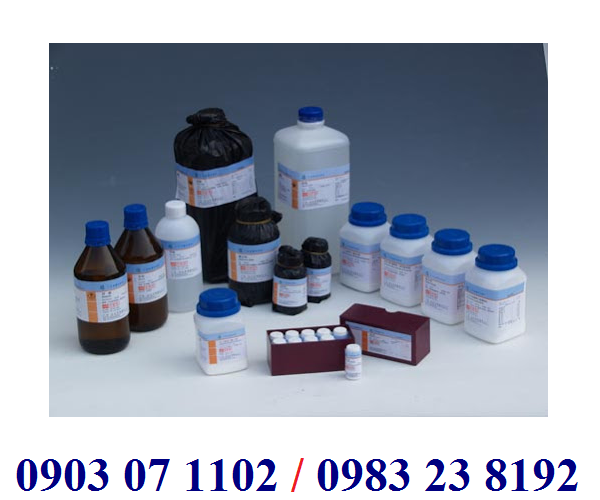The photograph showcases a detailed array of medical or scientific bottles placed on a white surface that transitions into a blue gradient background towards the center. The entire image is framed by a white border, with blue text at the bottom reading "0903071102/0983238192." The collection includes a variety of bottles, all adorned with white labels marked by a blue banner at the top. Among the assortment are:

- Two brown glass bottles with blue caps located on the far left.
- A series of white bottles with blue caps.
- A tall brown bottle with a dark cap.
- Several smaller brown bottles positioned in front of the larger containers.
- A distinctive brown cardboard box containing 10 small bottles with white caps.

The grouping features some bottles wrapped in black plastic and tied at the top, adding to the variety. Due to the resolution, the precise details on the labels are indistinguishable, but the uniform label design suggests pharmaceutical or scientific contents, such as chemicals or powders.